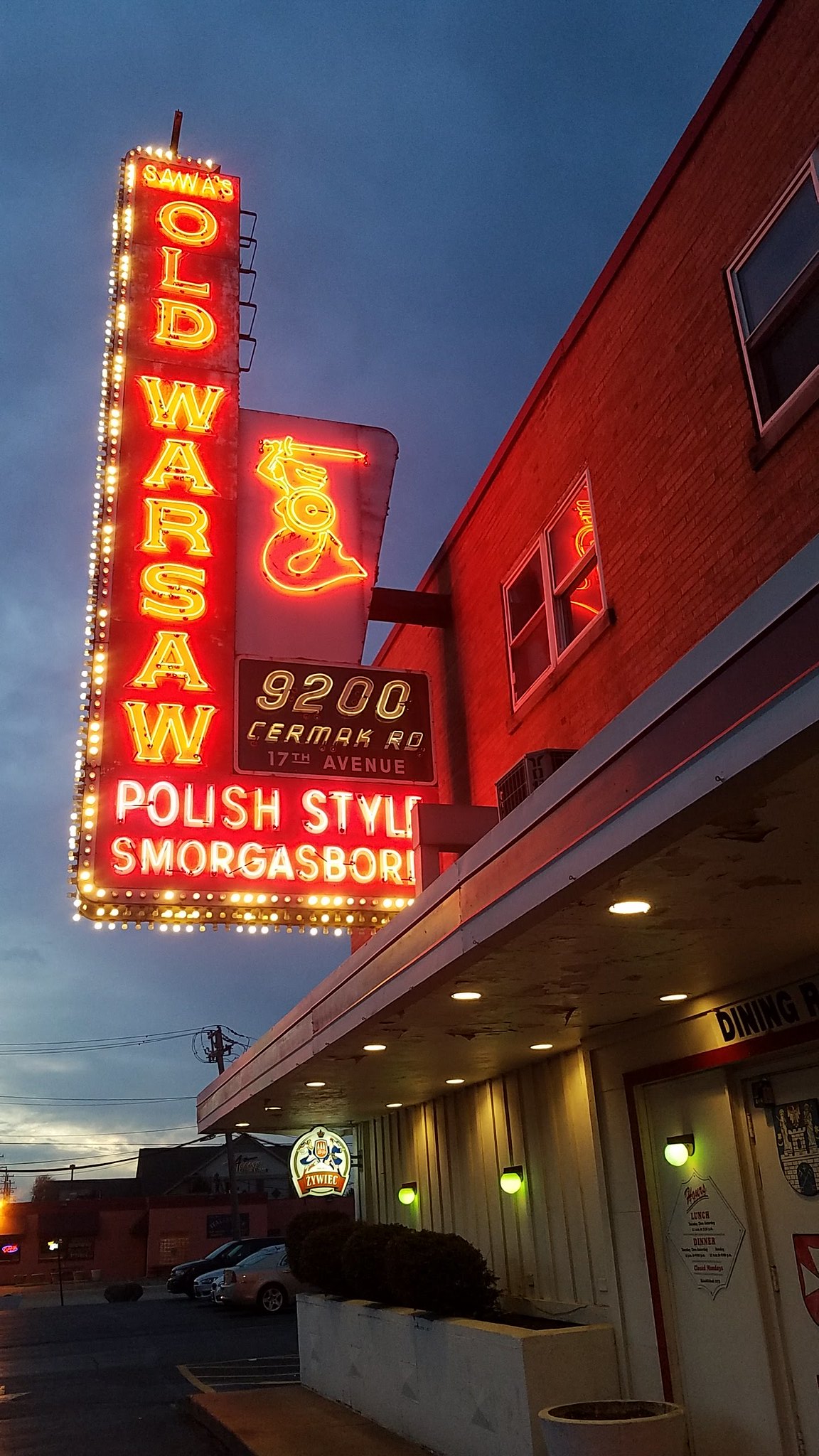The photograph, taken at dusk, showcases a close-up view of a two-story brick building with a prominent neon sign attached to it. The sky in the background is dark blue-gray, indicative of the sun having just set, with a few illuminated clouds on the horizon. The neon sign, shaped like the letter L, prominently juts out and up from the building. It features a red background with bright yellow neon lights running along its edges. The sign reads "Old Warsaw" vertically in yellow letters, and "Polish Style Smorgasbord" horizontally in bright white letters. Additionally, a black sign with golden numbers displays the address "9200 Cermak Road," indicating its location on the corner of 17th Avenue. The building itself has two white-edged windows on the upper floor, and a white door outlined in red on the bottom level, accompanied by three lights along the wall. Out front, a concrete planter houses three bushes, enhancing the entrance area. In the background, a small building, a few cars, and a parking lot can be seen, completing the scene.